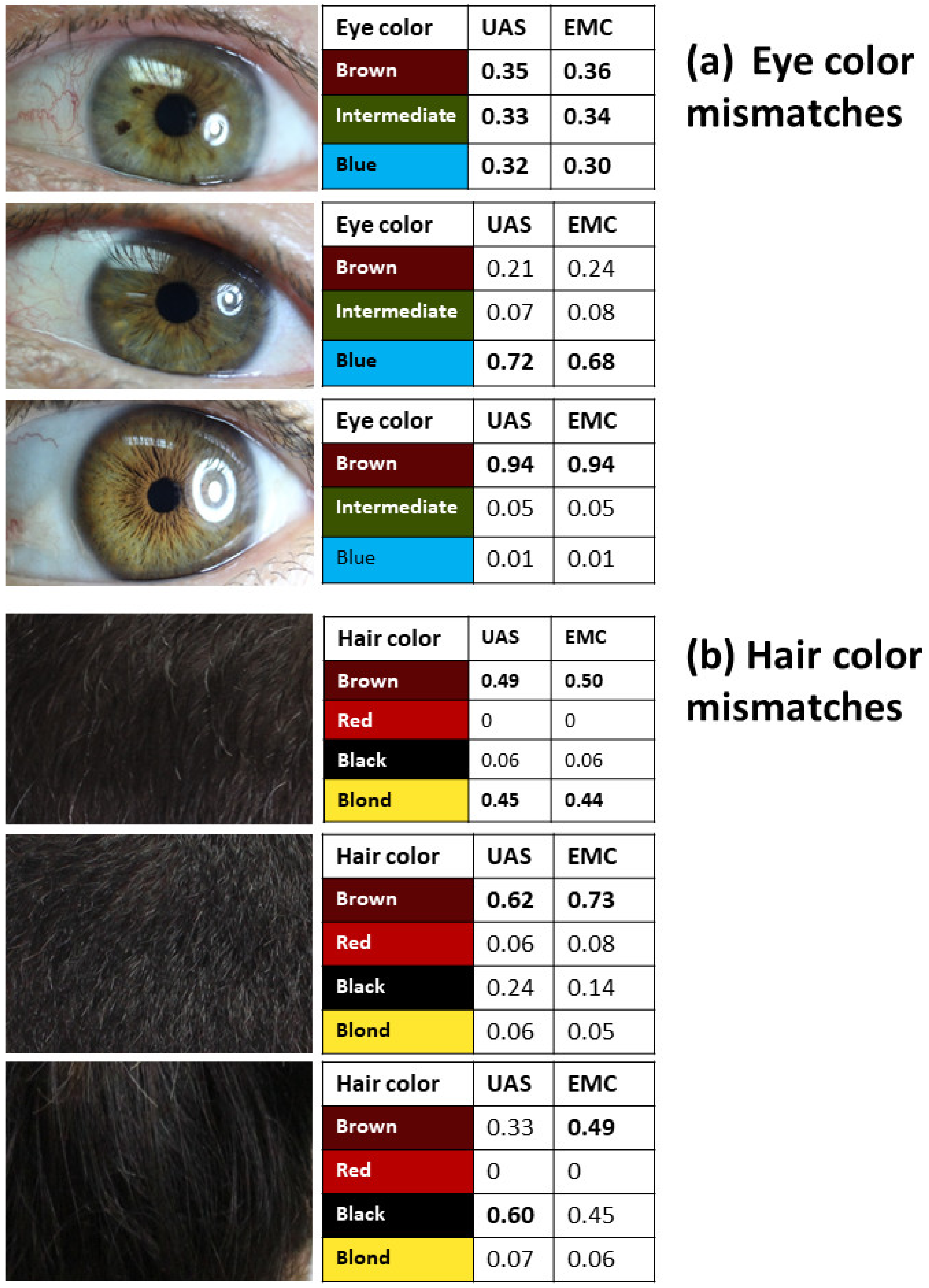The image comprises two vertically aligned charts, with the top chart focused on eye color and the bottom chart on hair color. 

In the eye color chart (Labelled "A: eye color mismatches"), there are three close-up photographs of eyeballs. To the right of these photographs, a chart displays the eye colors - brown, intermediate, and blue - in vertical sequence. Two columns labeled UAS and EMC contain numerical data corresponding to each eye color.

Beneath the eye chart is the hair color chart (Labelled "B: hair color mismatches"). Similar to the eye chart, it features three close-up photographs of dark-colored hair. To the right of these images, another chart lists hair colors - brown, red, black, and blonde - in a vertical arrangement. Like the eye chart, this one also includes two columns labeled UAS and EMC, populated with numbers pertaining to each hair color mismatch.

The detailed representation of color mismatches is consistent across both charts, showcasing how variations are documented and categorized under the UAS and EMC columns.